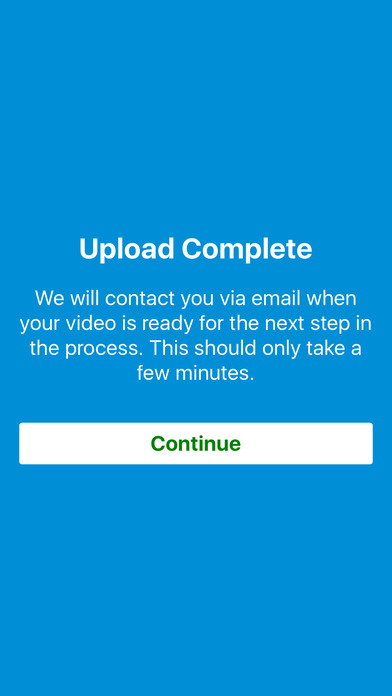The image appears to be a screenshot from a phone featuring a predominantly light blue vertical rectangle. Centrally positioned, there is bold white text reading "Upload Complete" just above the midpoint of the image. Directly below it, in a smaller and unbolded white font, the text states, "We will contact you via email when your video is ready for the next step in the process. This should only take a few minutes." Further down, a thin horizontal white rectangle nearly spans the entire width of the image, containing the word "Continue" in green text centrally aligned. All elements, including the text and the button, are centrally located, ensuring a straightforward and user-focused design. There are no additional details or elements within the screenshot.